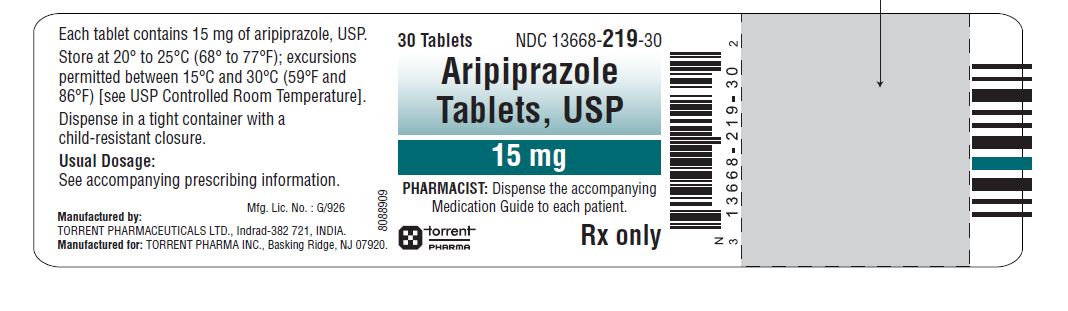In this image, a detailed pharmaceutical label is presented with the following information and design elements:

- **Main Label**: A large white label bordered in light blue.
- **Dosage Information**: On the left side, it reads: "Each tablet contains 15 mg of Aripiprazole, USP."
- **Storage Instructions**: The label specifies: "Store at 20 to 25 degrees Celsius (68 to 77 degrees Fahrenheit), with allowed excursions between 15 to 30 degrees Celsius (59 to 86 degrees Fahrenheit)."
- **Packaging Instructions**: "Control room temperature as per USP standards. Dispense in a tight container with a child-resistant closure."
- **Dosage Guidance**: "Usual dosage – see accompanying prescription information."
- **Manufacturing Details**: "Manufacturing License Number 61926. Manufactured by Torrent Pharmaceuticals Limited in India. Distributed by Torrent Pharma Incorporated, Basking Ridge, New Jersey."
- **Contents**: The label prominently notes: "30 tablets, NDC 13668-21930."
- **Highlight Boxes**:
  - A light blue box containing the text: "Aripiprazole tablets, USP."
  - A green box displaying the dosage: "15 milligrams."
- **Pharmacist Instructions**: "Pharmacist: Dispense the accompanying medication guide to each patient."
- **Manufacturer's Logo and Legal Info**: A small black box with a white "X" displaying the word "Torrent" and the notation "Rx only."
- **Barcodes**: There is a visible barcode on the side accompanying numerical data.
- **Additional Elements**:
  - A large blue box with a dashed line and a black arrow in the middle.
  - Additional portions of the barcode can be seen on the side of the label.

This detailed description should paint a vivid picture of the information and layout found on the pharmaceutical label.